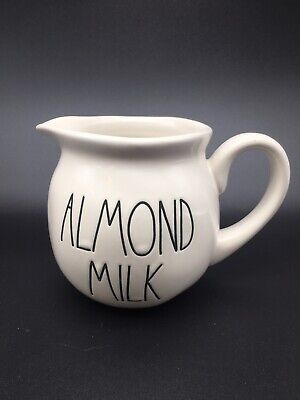The image showcases a small, trendy ceramic pitcher with a curved lip reminiscent of a mug. Crafted from porcelain with a cream-colored or eggshell white finish, the pitcher features a round, attached handle positioned to the right and a spout for pouring on the left. The words "almond milk" are inscribed in thin, stylish black font on the pitcher, giving a slightly puffy, textured feel to the text. The background transitions from a dark gray at the bottom to a lighter gray in the middle, then fades back to dark gray at the top, providing a gradient effect that frames the subject. The overall design, with its charming, imperfect lip and boutique-like aesthetic, suggests it could be a decorative piece found in a chic shop. The absence of objects for scale leaves its exact size ambiguous; it could be as small as a creamer or the size of a typical coffee mug.